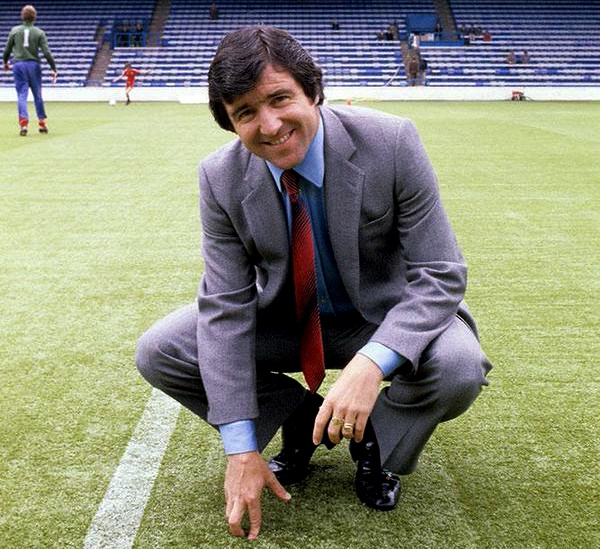The image captures a mid-20th-century scene set in a soccer stadium. At the front and center of the photograph, a man is squatting down on an artificial green turf, his left arm resting on his knee and his right hand touching the ground. He looks directly at the camera with a smile, dressed in a gray suit with a blue button-down shirt, a red tie, and shiny black leather shoes. His medium-length black hair is combed to the side, and a ring is visible on his left ring finger.

To his left, a white line on the turf is partially obscured by his body. In the background, spanning from left to right, are rows of empty blue and white seats, accentuated by a small white half-wall that separates the field from the stands. In the upper left portion of the image, two individuals are engaged in a casual soccer game. One, wearing a green shirt with the number one on it and blue pants, faces away from the camera, while the other, dressed in all red, appears ready to kick the ball. There are few people scattered in the stands, adding to the nostalgic and somewhat timeless quality of the scene.